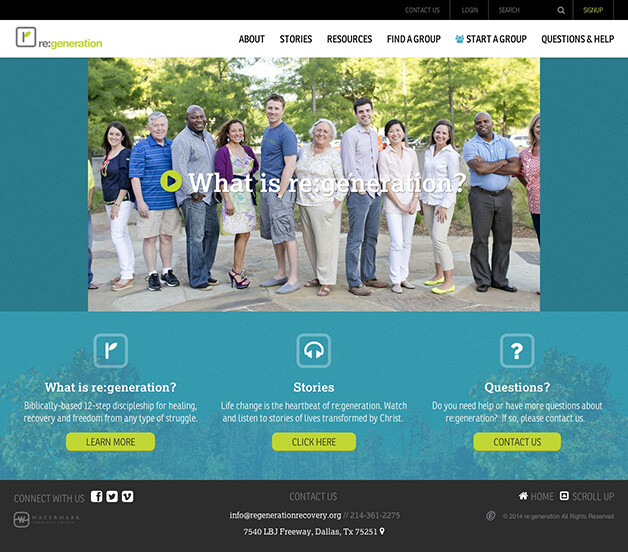The website features a black banner at the top with options like "Contact Us," "Log In," a search icon represented by a magnifying glass, and a "Sign Up" button in a greenish-yellow font. Below this, there is a white banner displaying a logo that consists of a square and a line with a leaf, accompanied by the text "RE:generation," where the word "generation" is in a lime green color. 

To the right of the logo, in black uppercase letters, are links labeled "About," "Stories," "Resources," "Find a Group," "Start a Group," "Questions," and "Help."

Further down, there's a section with a teal background featuring an image at its center. The image, which appears to be a video with a play button, depicts an outdoor scene with tall trees in various shades of green and glimpses of blue sky. In the foreground, there's a stone walkway with several people standing on it. Overlaid on this image is the question, "What is RE:generation?"

Underneath the image, against a lighter teal background, text reads: "What is RE:generation? Stories, Questions, Learn More, Click Here, Contact Us."